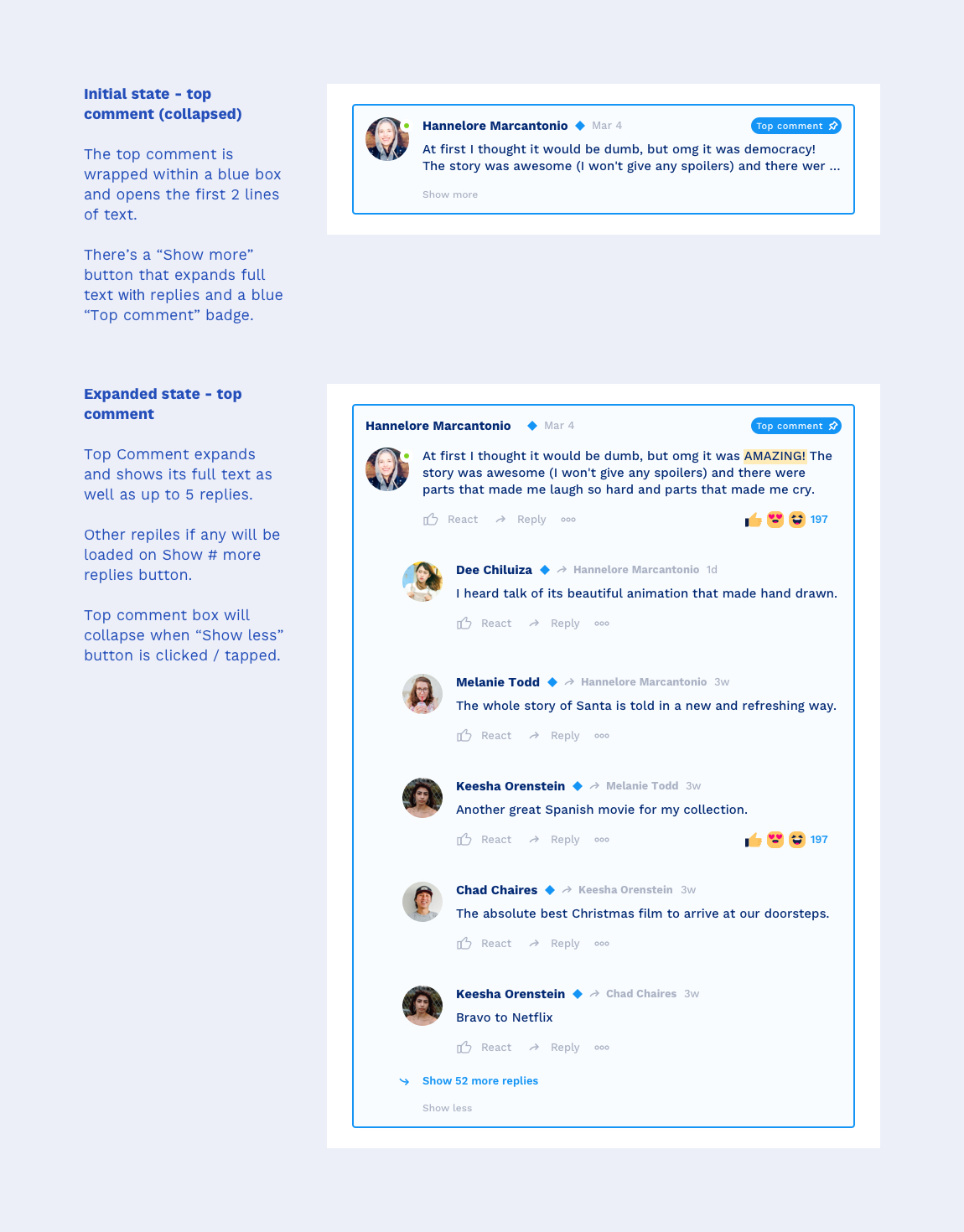In the image, there is a screen displayed on the left side that indicates the "initial state" wherein the top comment has been collapsed. This screen highlights the top comment which is enclosed within a blue box, showing only the first two lines of text. Below the comment, a "show more" button is available which, when clicked, expands to reveal the full text along with several replies. The top comment is identified by a blue "Top Comment" badge. 

The comment in question is by Hanalor Marcetonia, who begins with, "At first, I thought it would be dumb, but oh my god it was democracy. The story was awesome. I won't give any spoilers and there were," but is cut off at this point in the initial view. Hanalor's profile icon depicts a lady with blonde hair.

In the expanded state of the top comment, the full text of Hanalor’s comment is shown alongside up to five replies. Additional replies, if available, can be viewed by clicking a "show more" button at the bottom. There is also a "show less" button that collapses the comment back to its initial state. 

Hanalor's full comment reads, "At first, I thought it would be dumb, but oh my god it was amazing. The story was awesome. I won't give any spoilers and there were parts that made me laugh so hard and parts that made me cry." Among those who have replied to this comment are:

1. Dee Shazilla: "I heard talk of its beautiful animation that made hand-drawn."
2. Melanie Todd: "The whole story of Santa is told in a new and refreshing way."
3. Keisha Orenstein: "Another great Spanish movie for my collection."
4. Chad Charers: "The absolute best Christmas film to arrive at our doorsteps."
5. Keisha Greenstein: "Bravo, bravo to Netflix."

From these interactions, it appears that the comments are reviewing a Christmastime story, noting its beautiful hand-drawn animation, fresh take on the story of Santa, and overall emotional impact.